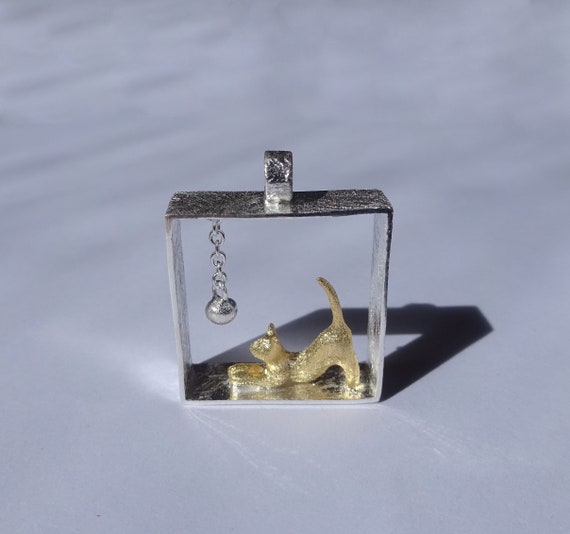The image showcases an ornamental piece that features a captivating scene encased in either crystal or glass. This decorative item intricately combines both gold and silver elements. At the base of the ornament, a golden cat is positioned with its back half raised, poised as though ready to pounce. Suspended from the top by a chain, a silver ball dangles, capturing the cat's attention. The silver ball, from certain angles, even resembles a cat's head with ears. The overall design suggests the piece could be hung, though it's not clear if there is a hole for hanging. The ornate craftsmanship and the playful scenario between the cat and the ball give the impression of an elegant and whimsical decoration.